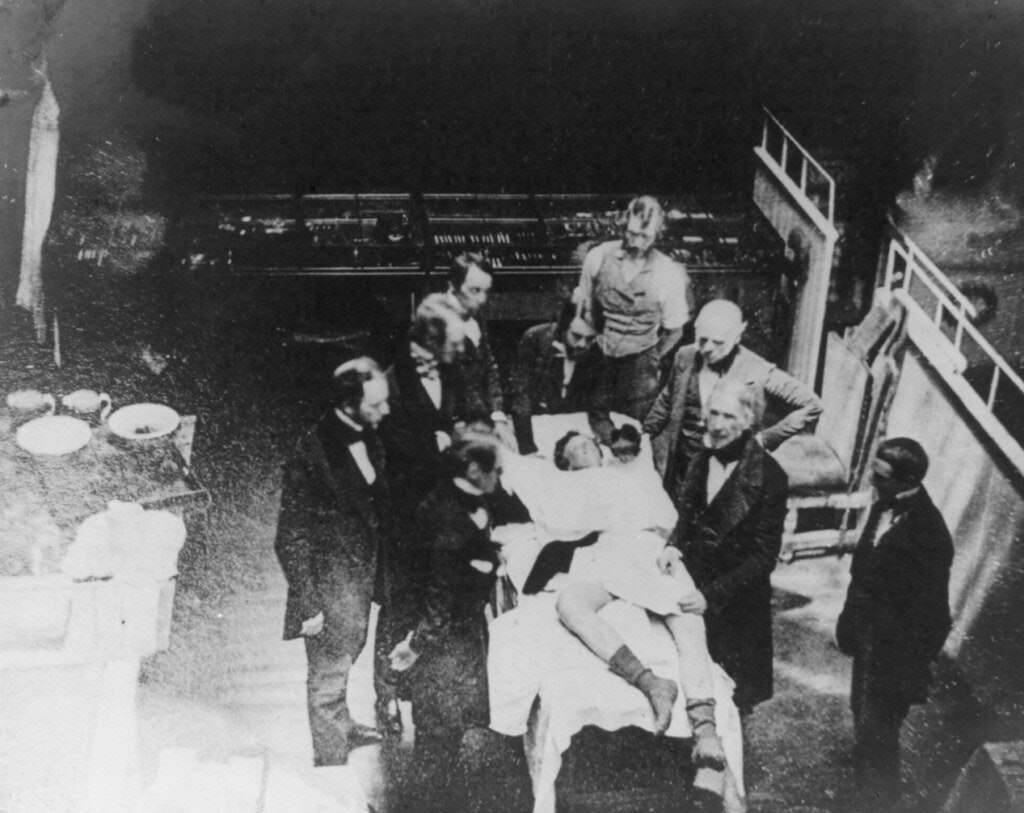This black and white aerial photograph, likely from the late 1800s or early 1900s, captures a grainy yet detailed scene in an operating theater. At the center, a patient, who appears to be either a gentleman or a lady, is lying on a small bed covered in white sheets. They are wearing dark tall socks and seem to be unconscious. Surrounding the patient are nine men, presumably doctors, the majority dressed in suits with black ties, though one at the back has removed his jacket. A man standing behind the patient's head is placing his hands under the patient's shoulders, while another man, positioned to the right of the patient, is looking up towards the camera. To the right of the scene are freestanding privacy dividers or curtains. The far side of the room features a control board, and the left side has assorted medical bowls or pans, suggesting the presence of surgical instruments.